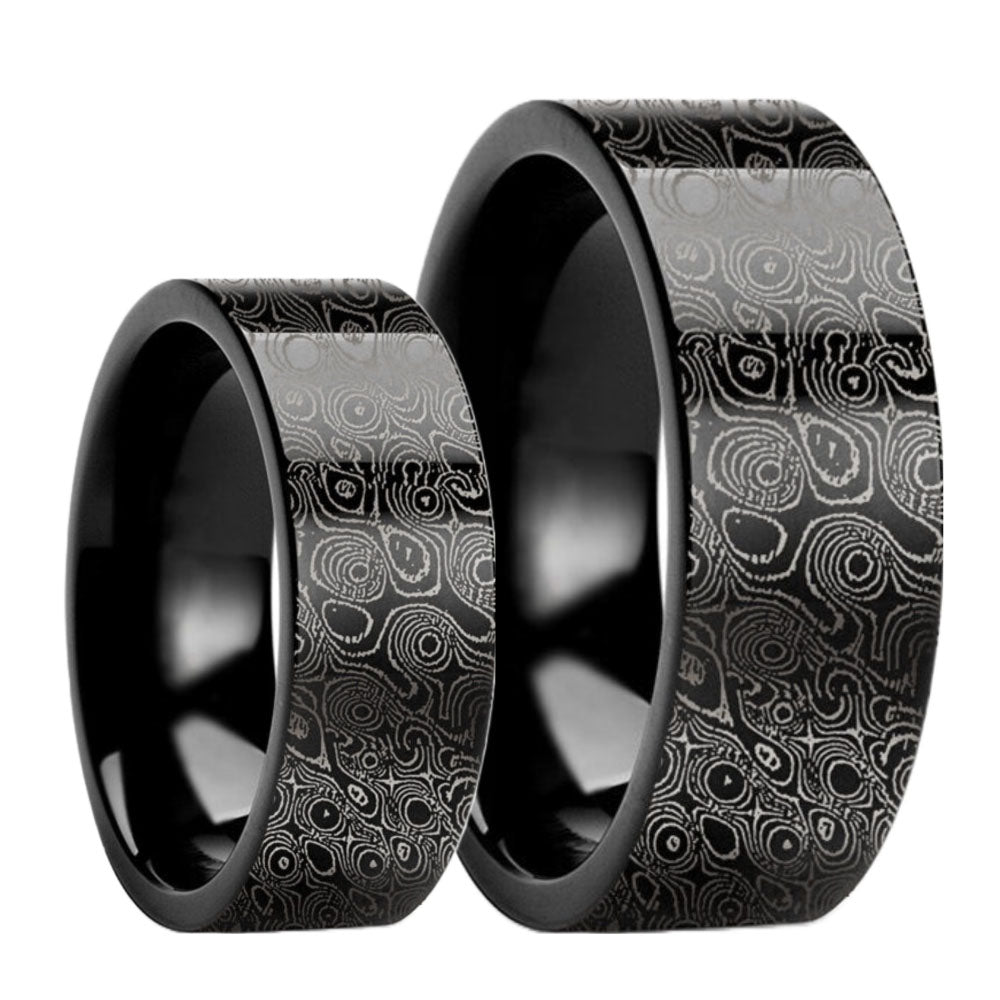The image features two black, shiny objects, resembling either rings or bowls, positioned on their sides against a solid white background. The larger object, on the right, is significantly bigger than the one on the left—almost half again its size. Both objects are adorned with intricate swirl-shaped patterns in light silver or gray, giving them a marbled appearance. The designs create a fingerprint or paisley-like effect around their exterior edges. Despite the uncertainty of their exact nature, the glossy, ridged surfaces and detailed patterns make the objects visually striking against the stark white backdrop.